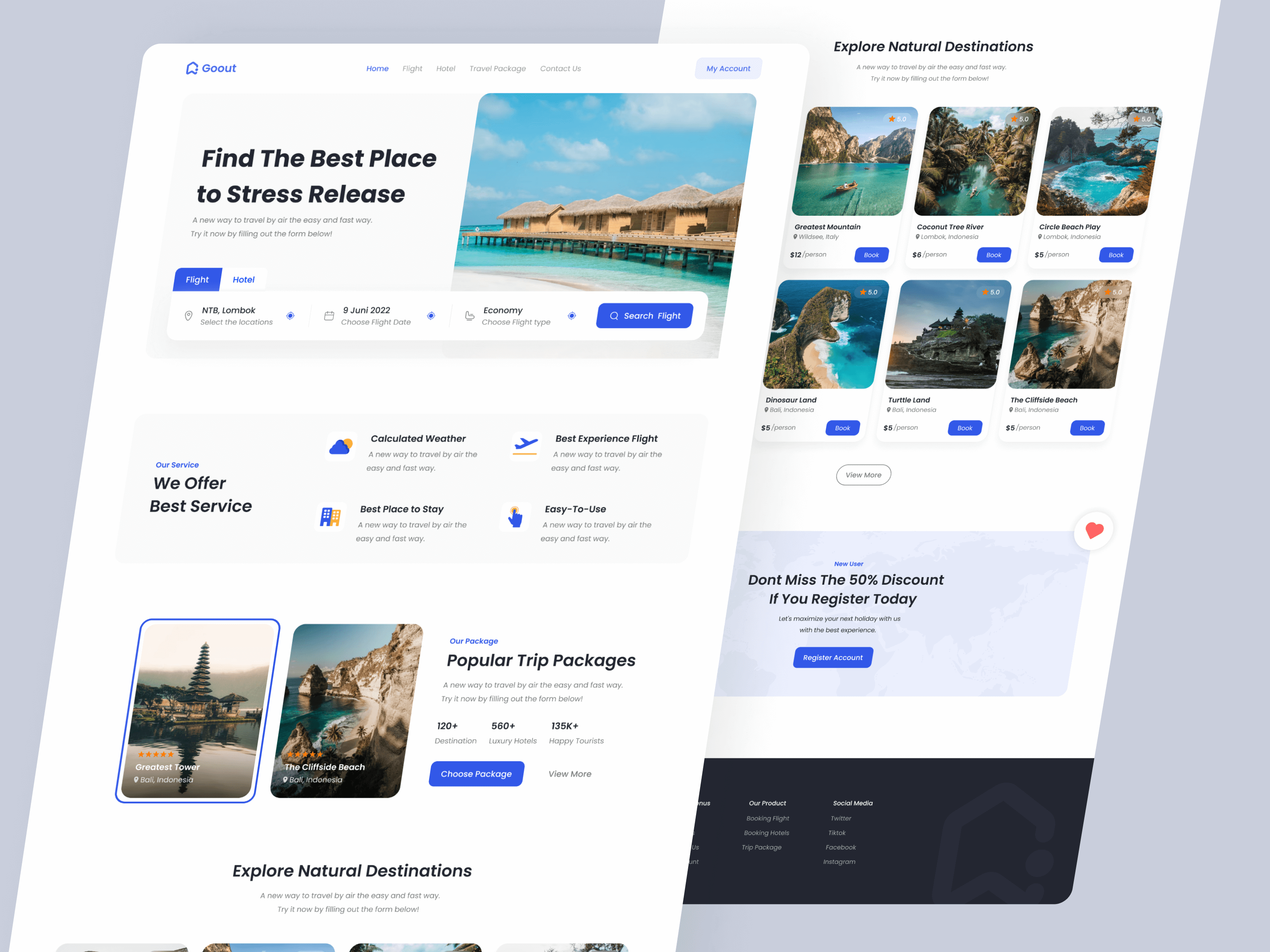This detailed descriptive caption encapsulates the given voice-described image:

---

The image is a screenshot of the travel website "Go Out." On the left side, the "Go Out" logo is prominently displayed. The image shows two different webpage sections, slightly angled to the right and overlapping towards the left. 

On the foremost webpage, the top navigation bar includes tabs labeled Home, Flight, Hotel, Travel Packages, and Contact Us. To the right of this navigation bar is a blue button labeled My Account. Below the navigation bar, there is a large image of hut-style villas situated over clear blue water, with the overlay text "Flight and Hotel." Currently, the "Hotel" tab is selected. The screen displays a series of options: an empty text field labeled “N-T-B-L-O-M-B-O-K,” followed by prompts to select the location, choose the flight date (set to June 2022), and select the flight type (set to Economy).

Beneath these options, there's a section listing various service highlights: "We offer the best service," "Calculated Weather," "Best Travel," "Best Experience Flight," "Best Place to Stay," and "Easy to Use." 

The bottom section of the screenshot showcases a variety of travel destinations.

---

This reformulated caption offers a comprehensive and structured overview of the elements present in the original image, enhancing clarity and detail.